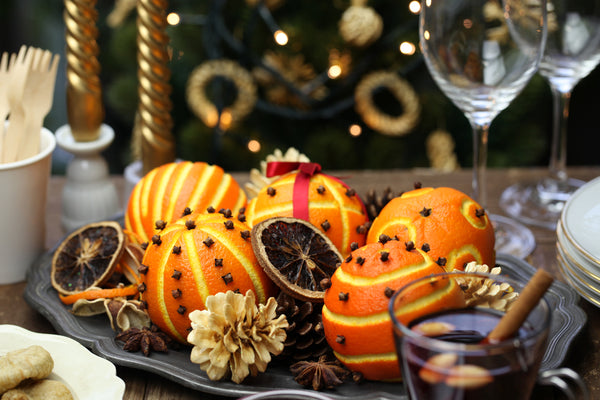In this close-up photograph, a beautifully arranged silver platter takes center stage on a wooden dining table set for a festive holiday gathering. The platter features five large navel oranges, each artistically carved with intricate patterns like stripes, checkers, circles, and spirals. Small, star-shaped cloves are meticulously stuck into four of these oranges, enhancing the decorative designs. Surrounding the vibrant oranges are an assortment of white and brown pinecones, dried orange slices, and a single orange wrapped with a red ribbon and bow. The table is further adorned with elegant golden taper candles, stacked plates, a glass of cider with a cinnamon stick, and empty wine glasses, alongside some plastic forks and a white cup. In the softly blurred background, golden lights and ornaments on a Christmas tree add a warm, festive ambiance, making it evident that this image captures the essence of a holiday party.